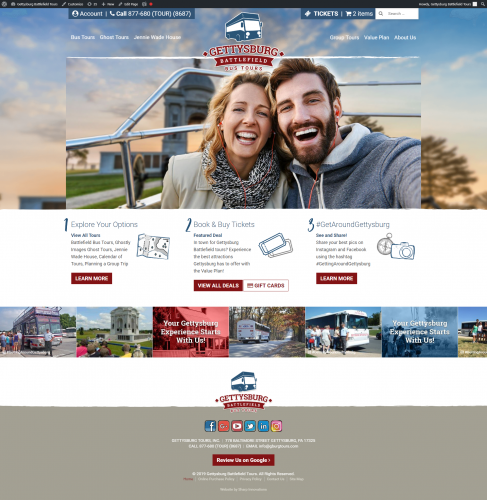This image appears to be a slightly blurry, small screenshot likely taken from a laptop. The primary structure is a square format, prominently featuring text and images that seem to relate to Gettysburg Battlefield Bus Tours.

From the upper left-hand corner to the upper right-hand corner, there is an illegible black stripe. Below this, the next row of text begins with the word "Account" and includes a phone number, "Call 877-680-TOUR." 

Centered in the image is a picture of a blue and white bus with the text "Gettysburg Battlefield Bus Tours" imprinted on it. Above this image, there's a mention of "Tickets" followed by "Two items."

In white text, several navigation tabs are listed, potentially including options like "Bus Tours," "Ghost Tours," "Jennie Wade's House," "Value Plan," and "About Us."

Dominating the central part of the image is a large photo featuring a light-skinned couple. The woman has blonde hair, and the man has brown hair along with a brown mustache and beard, giving him a distinctly 1860s Civil War appearance. They're dressed in winter clothing, and the backdrop showcases the Gettysburg Battlefield.

Towards the bottom of the image, a three-step process is outlined: "1. Explore Your Options," "2. Book and Buy Tickets," "3. Get Around Gettysburg." Accompanying these steps are red buttons designed for purchasing tickets. 

Finally, the bottom of the screenshot features social media links and additional thumbnail images seemingly intended to further assist users.